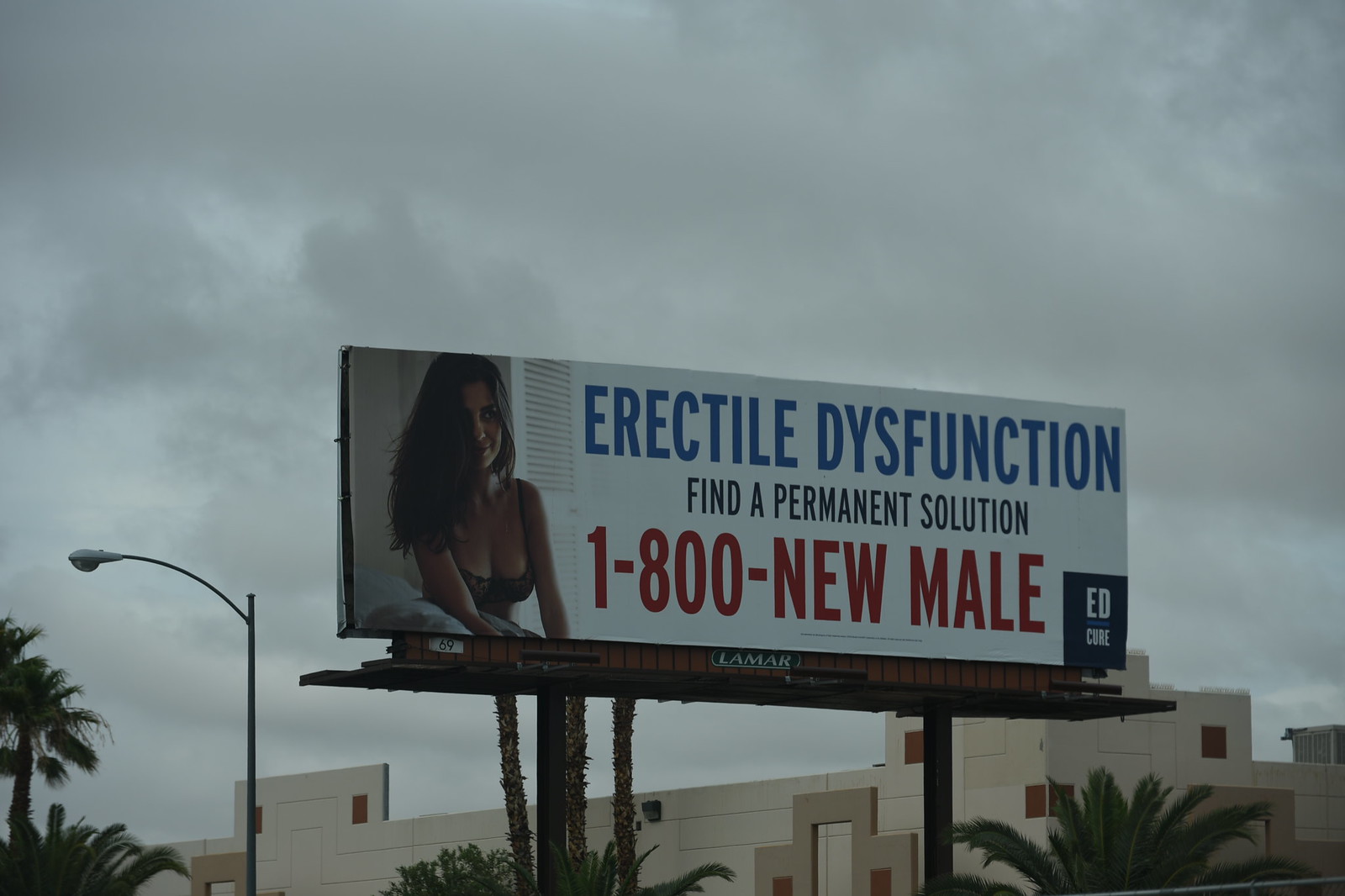This photograph captures an overcast day in a hot climate, possibly near a beach. Central to the image are several tall palm trees and a distinctive building made of large, white stone tiles that give it a striking resemblance to giant kitchen tiles. This building appears to be under construction or perhaps an art installation as it lacks a roof. To the left of this structure, a large, platform-mounted billboard dominates the scene. The billboard displays a striking advertisement featuring a woman with long brown hair dressed in a bra. Beside her image, large blue letters read "ERECTILE DYSFUNCTION," followed by smaller black-lettered text that says, “find a permanent solution.” The advertisement concludes with a prominently featured phone number in red: "1-800-NEWMAIL." Additional elements in the photograph include a few streetlights and the overall grey, overcast sky, adding a somber tone to the bustling setting.